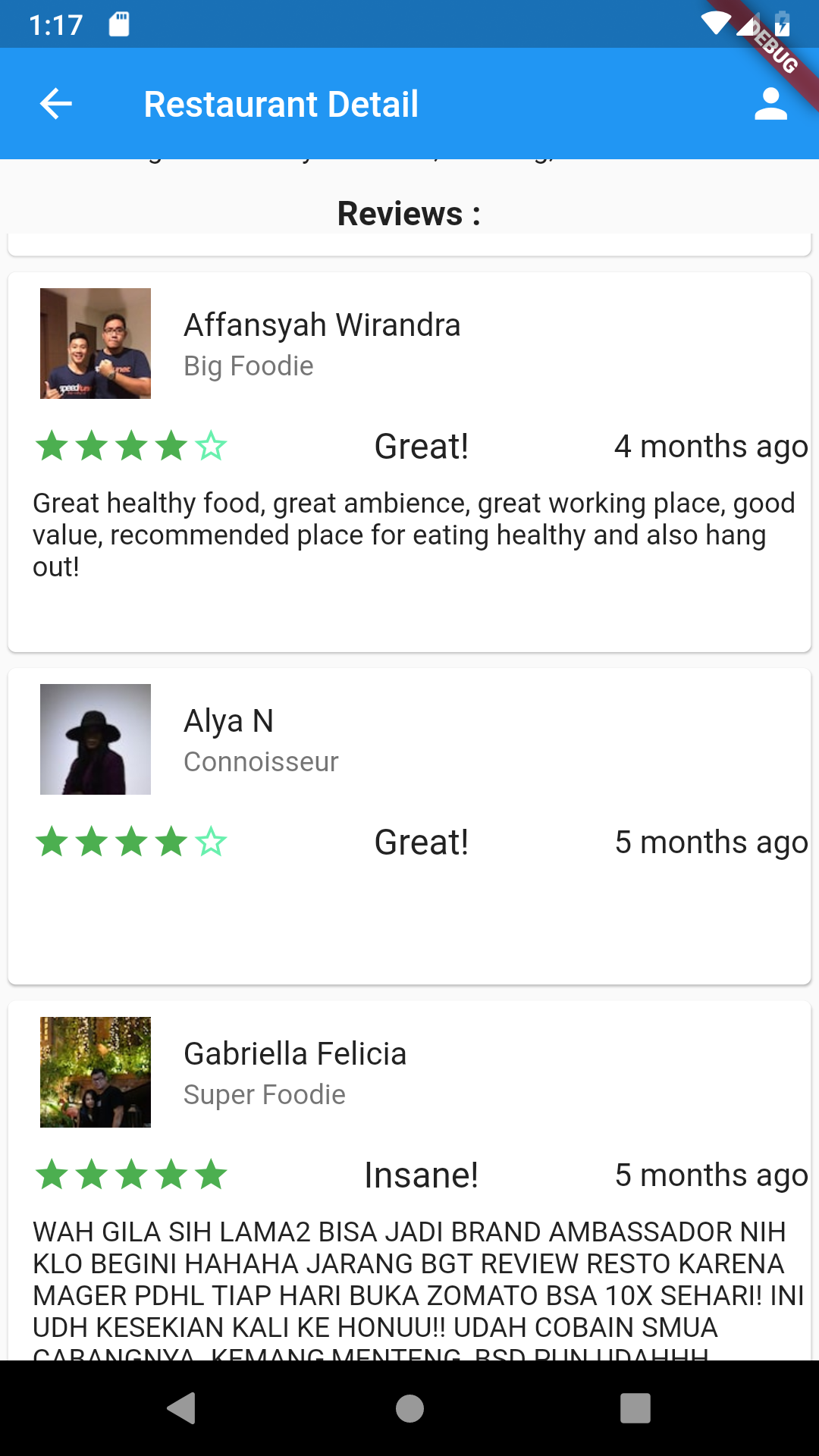A screenshot from a smartphone shows detailed restaurant reviews under the "Restaurant Detail" section. The phone's clock displays the time as 1:17. Three reviews are visible, each accompanied by a profile picture. The top review holds a four-star rating and displays a headline of "Great." The profile picture for this review features two gentlemen with dark hair wearing the same t-shirt. The second review also provides a four-star rating with the headline "Great," and features a generic shadow profile picture, indicative of an anonymous or default user icon. The third review is rated five stars, with a headline stating "Insane." The profile picture for this review depicts a couple, with a taller gentleman and a shorter female, possibly indicating a romantic or familial relationship.